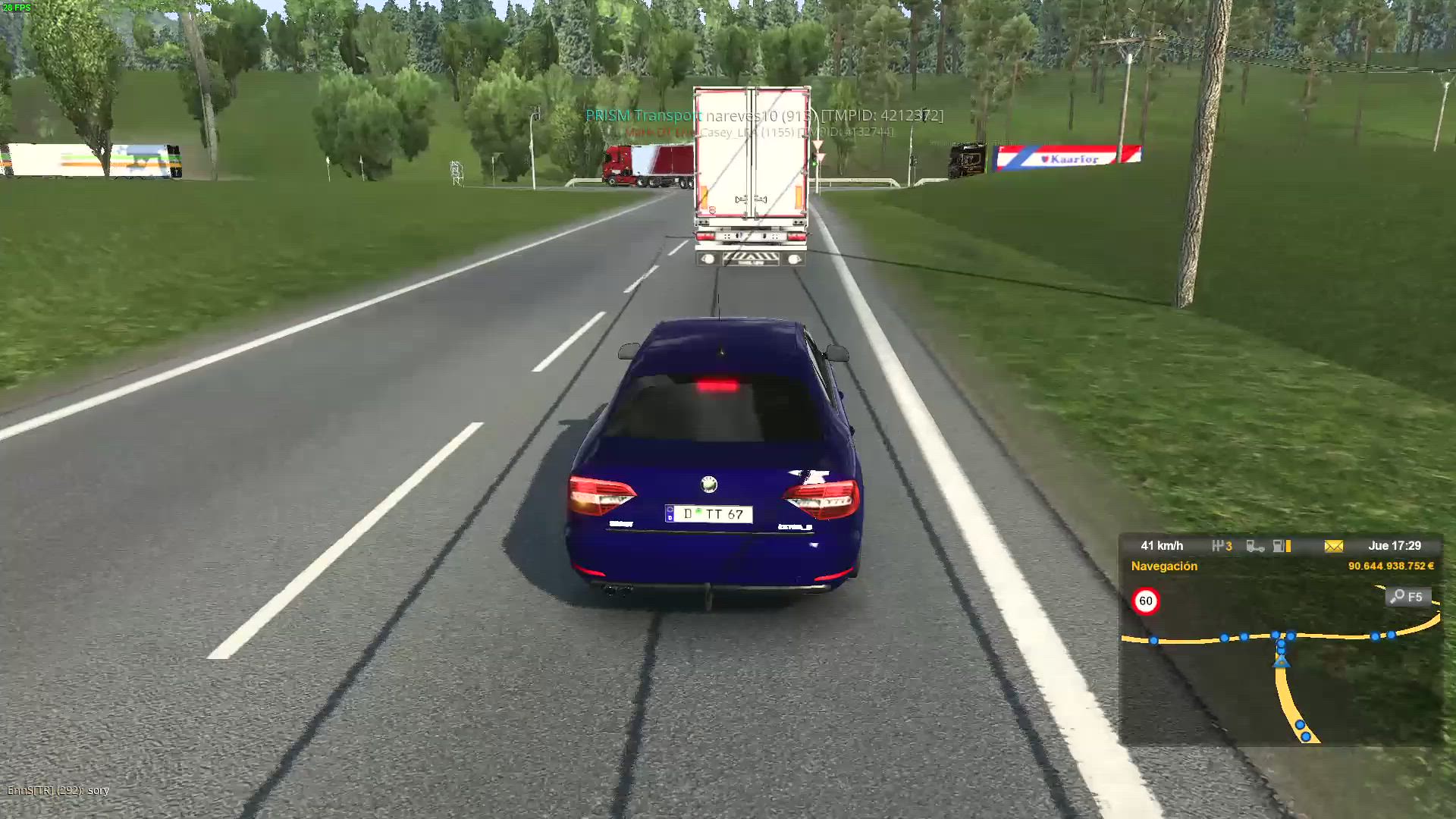The image is a 3D rendering of a gray, two-lane street with intermittent white dashes marking the lanes and bordered by solid white lines. The street is lined on both sides with grass and scattered trees, which extend into the background along with utility poles. The sky is depicted as blue, enhancing the daytime setting.

In the immediate foreground, there's a dark blue sedan with red taillights and a red brake bar at the top center of the rear windshield. The sedan, though its license plate is unreadable, appears to be driving away from the viewer. Directly ahead of the sedan is a white trailer truck. Further up the road, rounding a left curve, is a red and white trailer truck. In the distance to the left, another trailer truck with a white body and a yellow stripe on its side is visible.

The lower right corner of the image features a rectangular navigation map display. This small map, reminiscent of in-car GPS systems, shows a yellow T-shaped road with blue dots indicating navigation points. Text on the map is partially blurry but suggests a speed of 41 kilometers per hour on January 17th, reading 'JUE 1729' at the top. Additionally, a 66 is encircled in red within the map interface.

Overall, the image provides a detailed and immersive depiction of a driving scenario in a verdant, semi-urban environment, capturing both the road details and the vehicles in a vividly realistic manner.